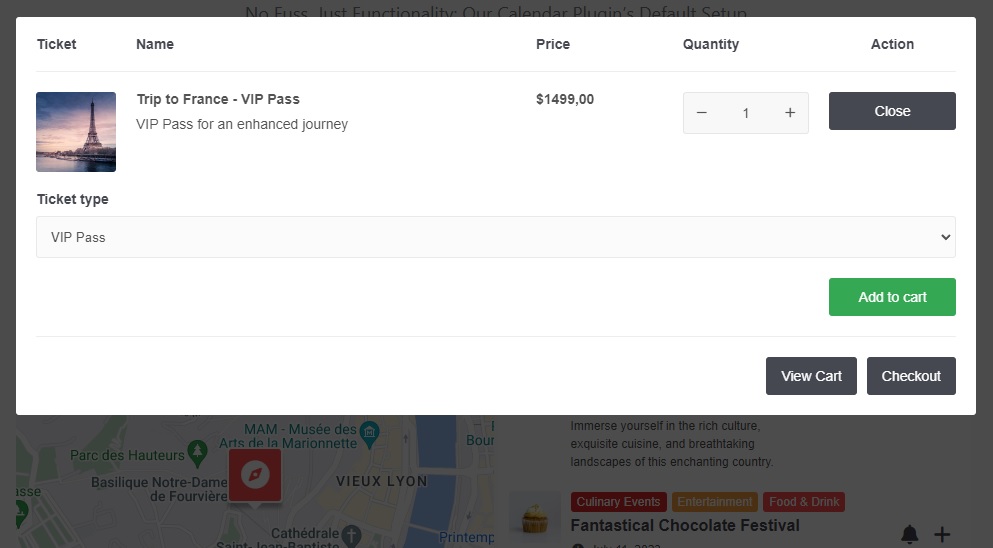A screenshot of a travel website is displayed, highlighting a specific package selection for a trip to France. An active dialog box shows various details about the chosen package, organized into five columns labeled: Ticket, Name, Price, Quantity, and Action. The selected trip prominently features a small thumbnail image of the Eiffel Tower, suggesting a French destination. Further beneath the image, details about the selected item reveal it as a "VIP Pass for an Enhanced Journey" priced at $1,499, with a quantity of one. Users have the option to close this selection window.

The ticket type displayed is the VIP Pass, confirming the selected option. Beneath the package details lies a green "Add to Cart" button with white text for users to add the package to their shopping cart. Additionally, there are two more buttons below: one on the left labeled "View Cart" and another on the right labeled "Checkout," enabling users to either review their cart contents or proceed directly to checkout.